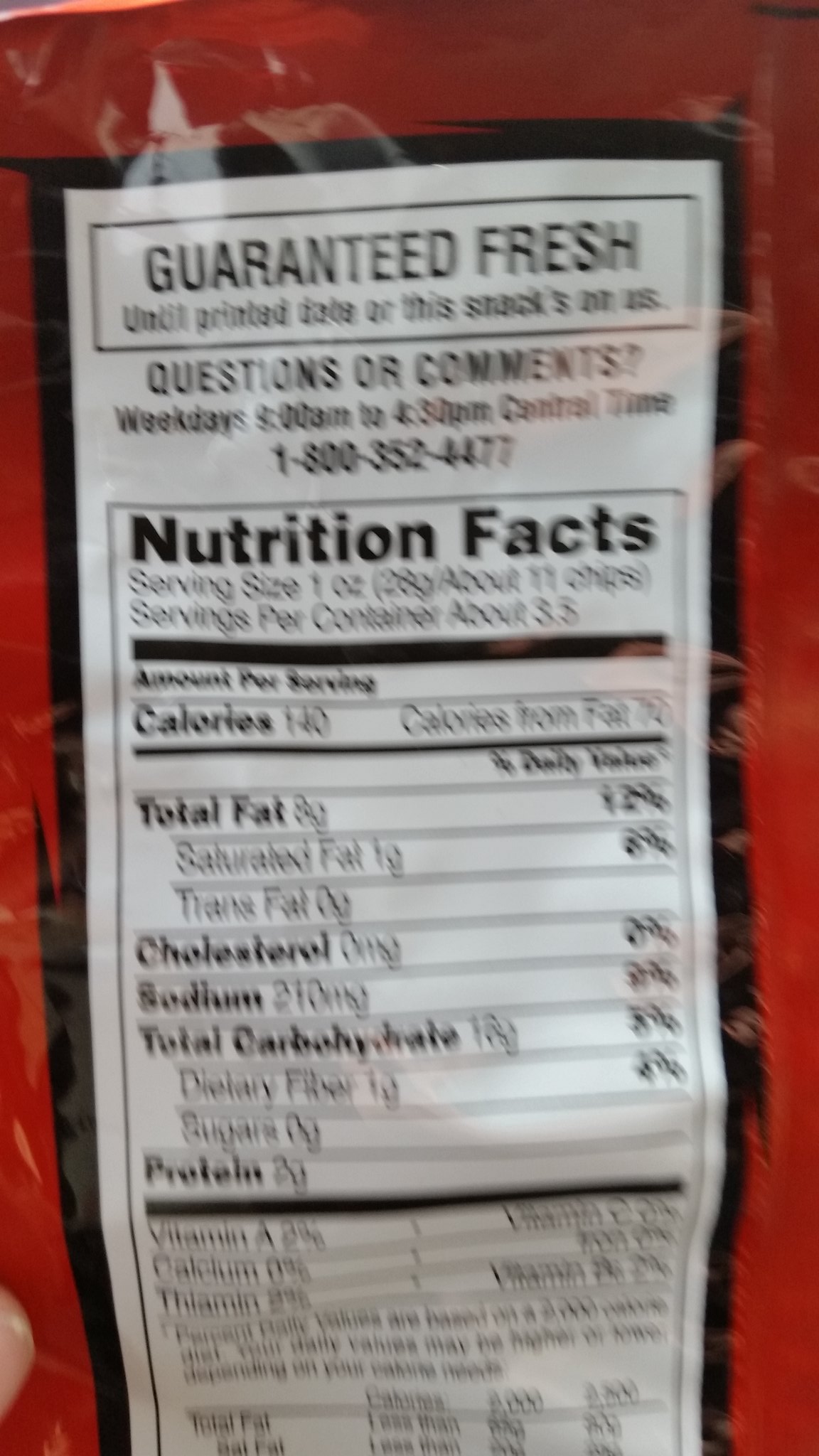The image depicts the slightly blurry back of a red, shiny bag, resembling a bag of chips, potentially Doritos. A person's finger is visible at the bottom left, holding the bag. The nutritional facts are displayed within a white box bordered by black. Key details from the label include: "Guaranteed fresh until printed date or the snack is on us. Questions or comments? Weekdays 9 a.m. to 4:30 p.m. Central Time, 1-800-352-4477." Nutritional information includes a serving size of 1 ounce, about 11 chips, with approximately 3.5 servings per container, totaling 140 calories per serving. The label indicates 70 calories from fat, 8 grams of total fat, 1 gram of saturated fat, 0 grams of trans fat, 0 milligrams of cholesterol, 210 milligrams of sodium, 18 grams of total carbohydrates, 1 gram of dietary fiber, 0 grams of sugar, and between 2 and 3 grams of protein, though the exact protein content is unclear due to the blurriness.